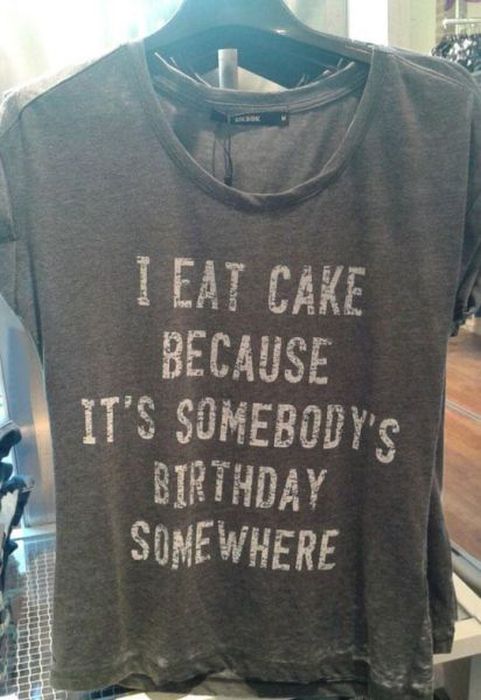The image depicts a dark grey, short-sleeved, round neck t-shirt, prominently displayed in a fashion shop, hanging on a black hanger. The t-shirt features a playful, distressed white font printed across the chest that reads, "I EAT CAKE BECAUSE IT'S SOMEBODY'S BIRTHDAY SOMEWHERE," all in capitalized letters. The t-shirt, with a laid-back, baggy fit, suggests softness and comfort. Below the t-shirt, there's a white shelf or tray with a lacquered top. The image also captures a glimpse of wooden brown flooring under the shelf and part of another clothing rack in the far right corner of the image, displaying black and white clothes. The top right corner behind the t-shirt shows the portion of a white pole with additional hangers.